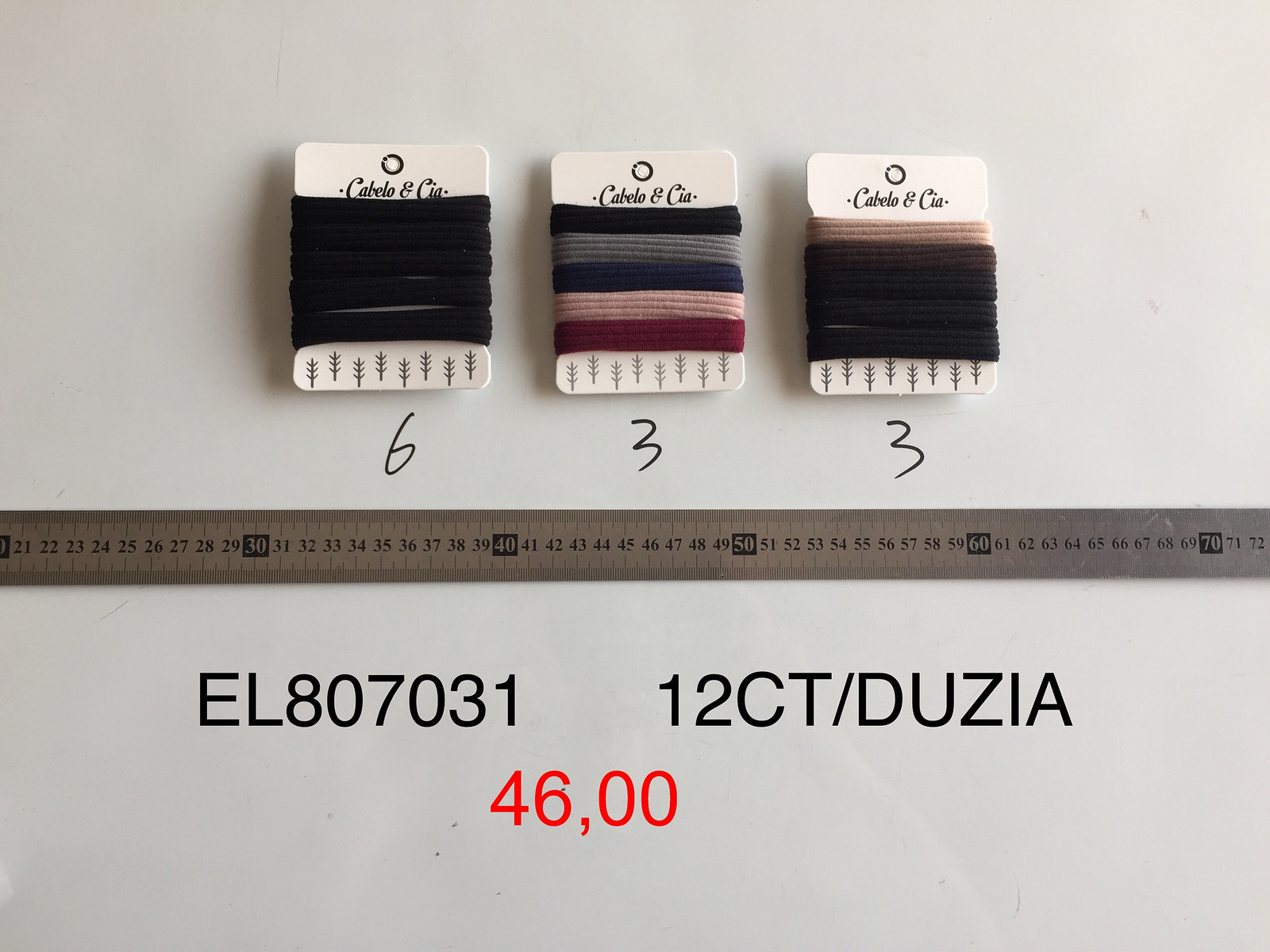This detailed photograph features a horizontal rectangle image against a white background, likely suggesting either a flat surface or items hanging on a wall. Dominating the top half are three cards displaying sets of scrunchie hair bands, labeled with "Cabello and Co." Each card is light beige with a metal circle for hanging. The first card on the left holds five black hair bands. The middle card presents a colorful assortment, featuring bands in black, gray, blue, pink, and maroon. The third card on the right has bands in tan, dark brown, and three shades of black. Below each card, handwritten in black font, are the numbers six, three, and three, corresponding to each set respectively. 

Intersecting the lower half of the photograph is a stainless steel tape measure running horizontally, marked with black text, scaling from 21 to 72 centimeters. Beneath the tape measure, in black text, are the product codes "EL807031" and "12 CT / DUZIA." At the very bottom, in red ink, the number "46,00" is prominently displayed.